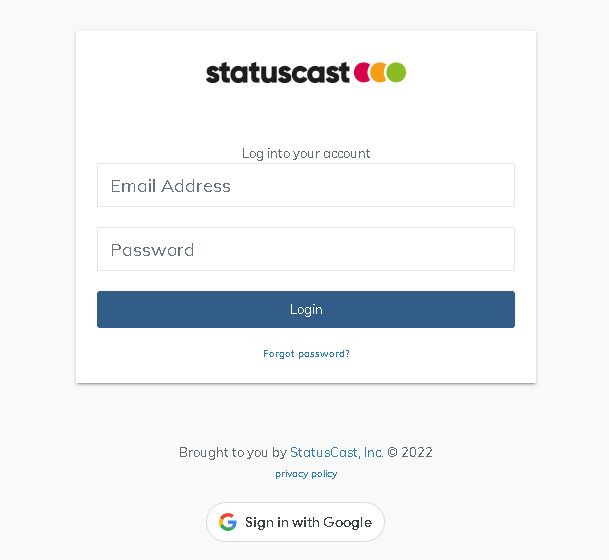A screenshot of a website featuring the "StatusCast" logo prominently displayed in bold black letters at the top. Adjacent to the logo are three circles colored red, yellow, and green respectively. The image has a minimalist white background. Below the logo, the text "Log in to your account" is written in black, guiding users to an entry field labeled "Email address." Beneath this, another input field is present for the "Password," marked similarly in black letters. 

Further down, there is a clickable blue button with the text "Log in" in white. Just below this button, the phrase "Forgot password?" appears as an interactive link in blue, complete with a question mark. The surrounding background of the webpage is a light gray shade.

At the bottom, the text reads "Brought to you by StatusCast Incorporated © 2022," with links to "StatusCast Incorporated" and their "Privacy Policy," both clickable and presented in blue. Additionally, the page includes an option to "Sign in with Google." This is displayed within an oval button, styled in black text with a multicolored Google logo (red, blue, green, yellow) adjacent to it.